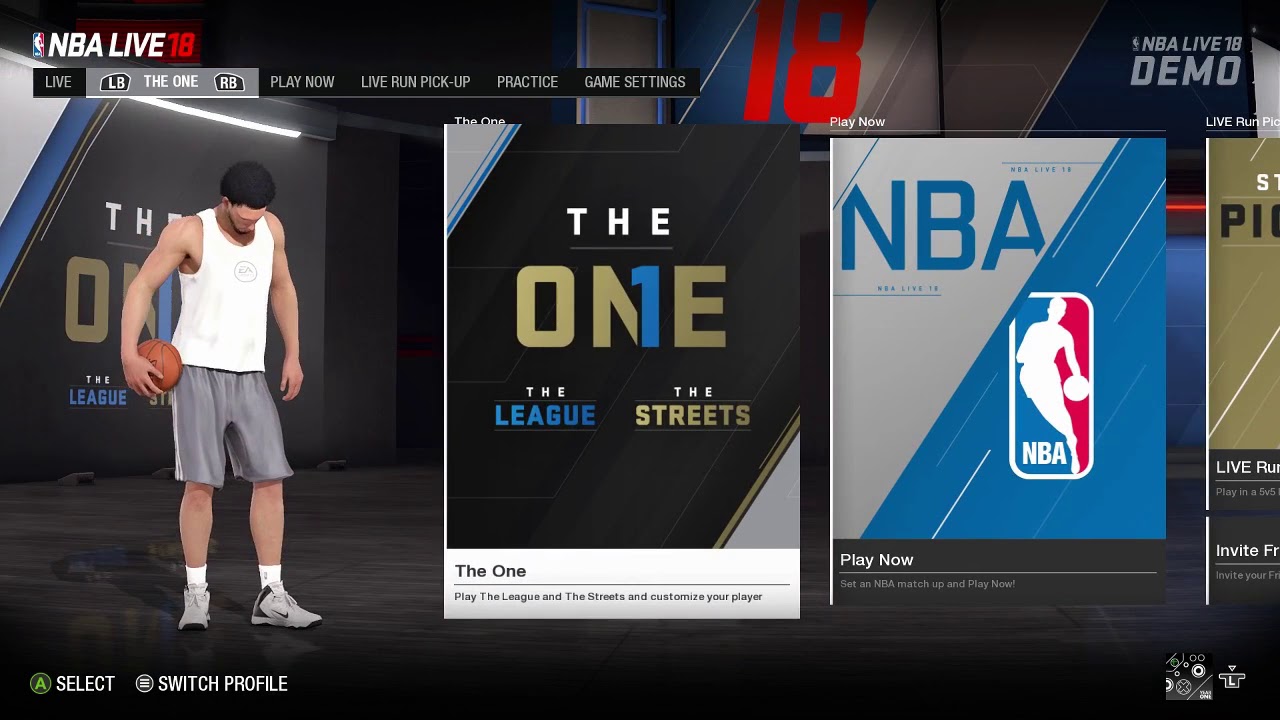In the upper left corner of the image, there's a gray box labeled "NBA Live," and another box titled "The One." Additionally, the screen displays options including "Play Now," "Live Run," "Pick," "Practice," "Game Sentence," and "NBA Live 10 Demo." Two smaller boxes feature more options, one of which reads "The One," "The League," and "The Streets," while the bottom part repeats "The One."

To the right, a gray and blue box prominently displays the NBA logo, depicting the iconic basketball silhouette. To the left of this logo, a basketball player is shown wearing a white tank top, gray shorts, and white Nike shoes, complete with the recognizable Nike swoosh.

At the bottom of the screen, a green circle reads "Select," and a gray circle indicates "Switch Profile." The setting features walls painted in a combination of white, blue, and black, with a fluorescent bulb hanging from the ceiling, providing illumination.